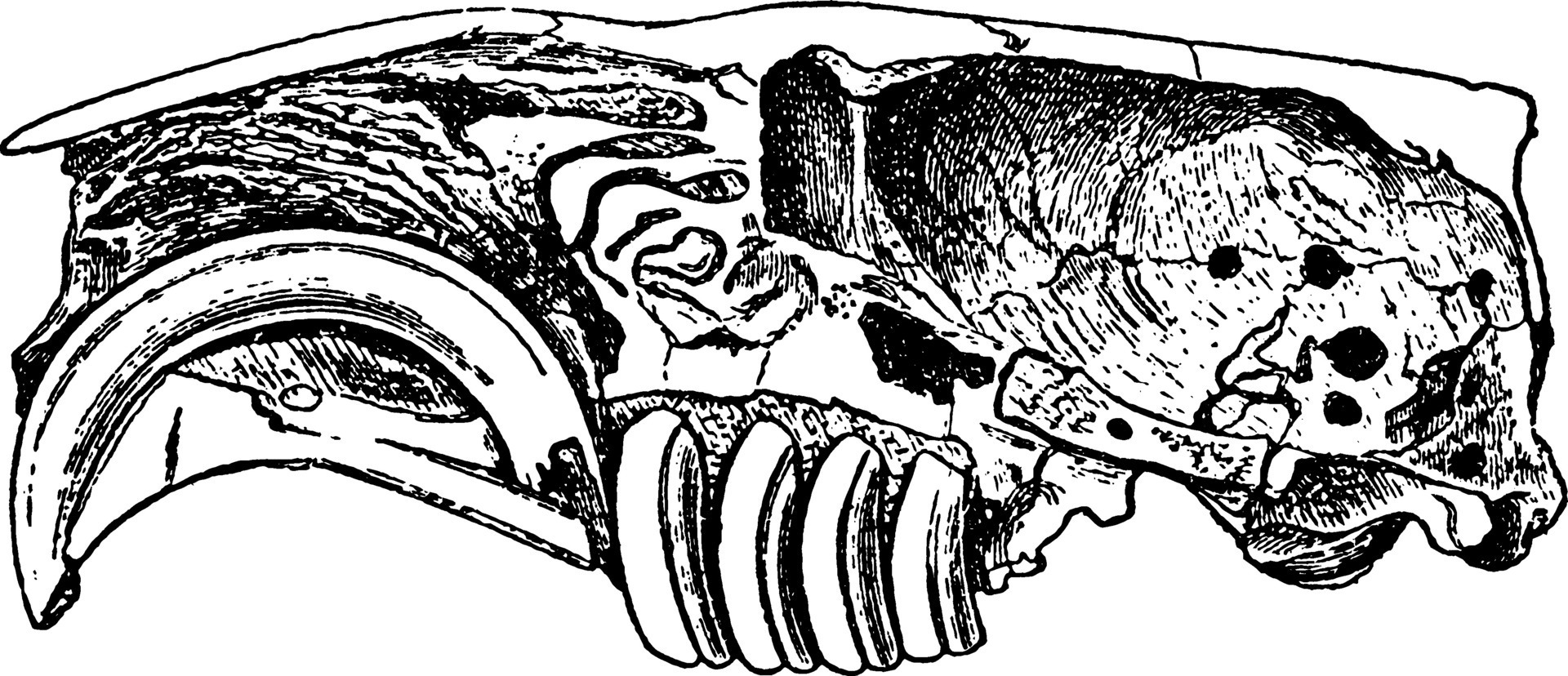The black and white illustration depicts a partially sliced-open side view of a skull, possibly of a rodent or rabbit, rendered in an ink style with shading. The image focuses on a smooth, curved piece extending outward from what appears to be a skull cavity, suggesting it could be teeth – specifically one prominent incisor and four molars located centrally behind it. The object features a ridge along the top, several holes, and cracks, contributing to its fragmented appearance. Despite its ambiguity, the image hints at a fossilized or archaeological find, characterized by jagged edges and a concave section, making it unclear whether it's a biological specimen, a bone fragment, or possibly even an ancient tool.